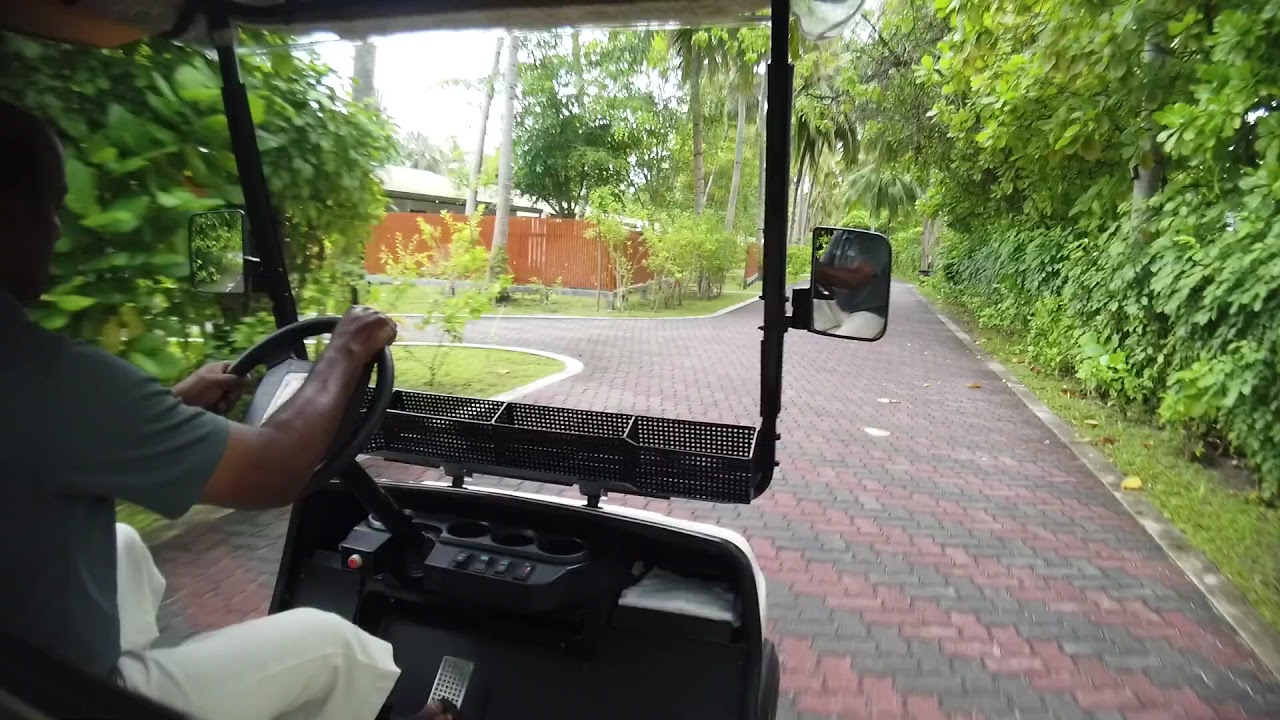In this image, a person is driving a golf cart down a diagonally patterned brick pathway composed of alternating dark red and dark gray bricks. The scene is set in a tropical environment, evidenced by the combination of palm trees on the left and large, verdant deciduous trees on the right, creating a lush green canopy overhead. The image perspective suggests it was taken from just behind or to the side of the driver, possibly from the back seat of the golf cart. 

The driver, a dark-skinned man, is wearing white pants and a gray short-sleeve t-shirt. The golf cart itself features a windshield and side mirrors. The front of the cart is visible along the left edge of the image, with the driver's side mirror partially obscuring the view down the path. 

To the left side of the path, there is an orange wooden fence enclosing a single-story building with a white or light-colored roof. The pathway in front of the cart splits, with one additional segment veering off to the left, hinting at an intersection. The overall setting suggests a serene, car-free zone, possibly within a resort or residential area, adding to the tranquil and tropical ambiance.